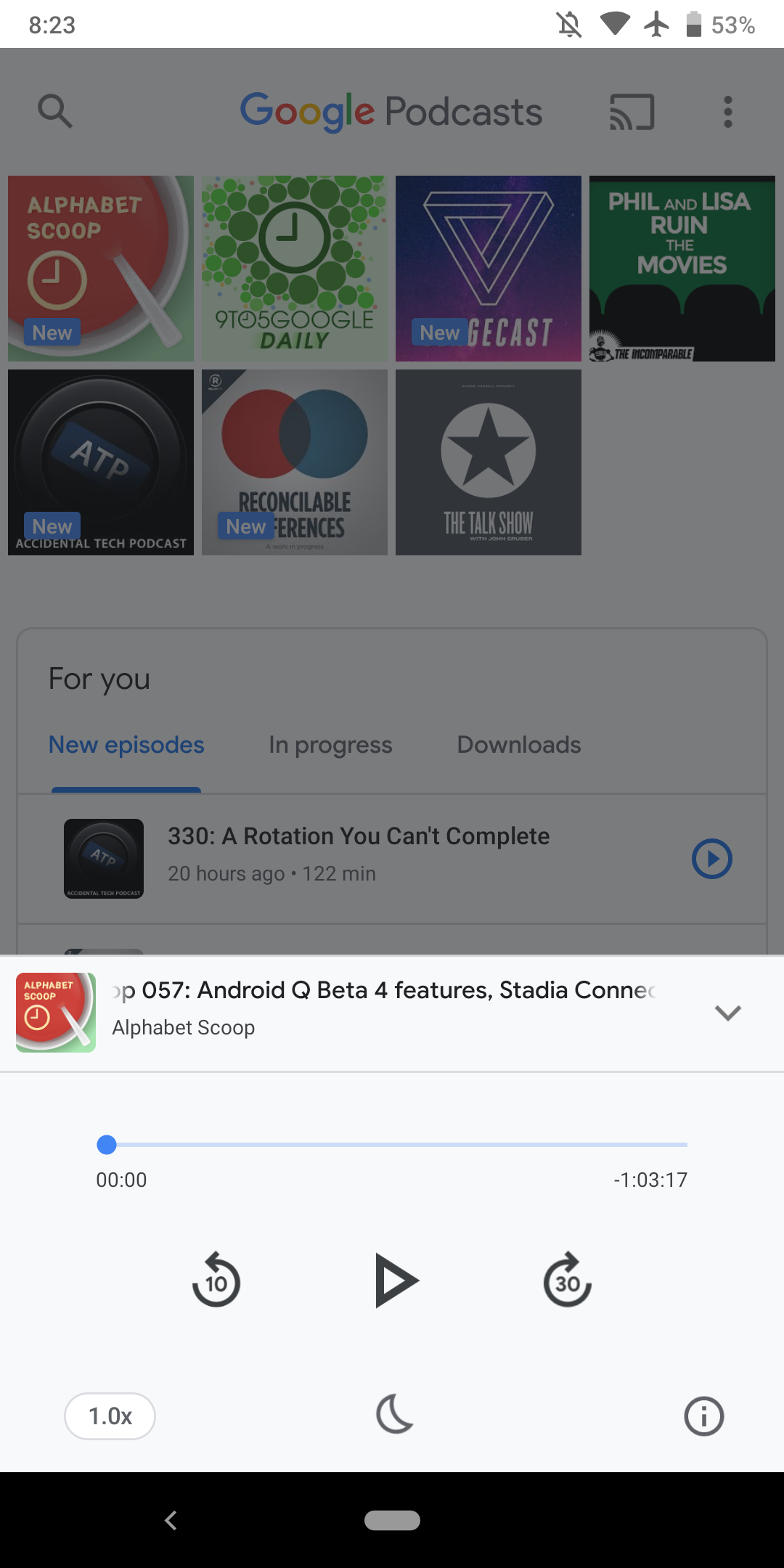The image depicts a dark-themed interface of the Google Podcasts app, displayed on a mobile phone. At the top of the screen, the Google logo is prominently featured, with its signature blue, red, yellow, and green letters. Below, "Podcasts" is written in black.

The status bar at the top shows the phone's battery life at 83%, with it being in airplane mode and the current time at 8:23. The signal strength is indicated as strong.

The main content area displays various podcast covers. The first visible cover, titled "Alphabet Soup," includes an image of soup with a clock in it. Another podcast, showcased with a green cover, is named "Google Daily." A purple podcast cover mentions "Phil and Lisa Ruined the Movies," featuring silhouettes of a man and a woman. Additional podcast titles include "ATP," "Reconcilable Differences," and "The Talk Show."

The screen also highlights different sections such as "For You," as well as categories like "New Episodes," "In Progress," and "Downloads." At the bottom of the screen, which transitions to a white-background interface, there's a section on "Android Beta Features" and "Stadia Connection," with a clickable image of "Alphabet Scoop" for easy access to start listening.

In summary, the screenshot effectively showcases the user interface of the Google Podcasts app with detailed descriptions of podcast covers, functional sections, and device status.